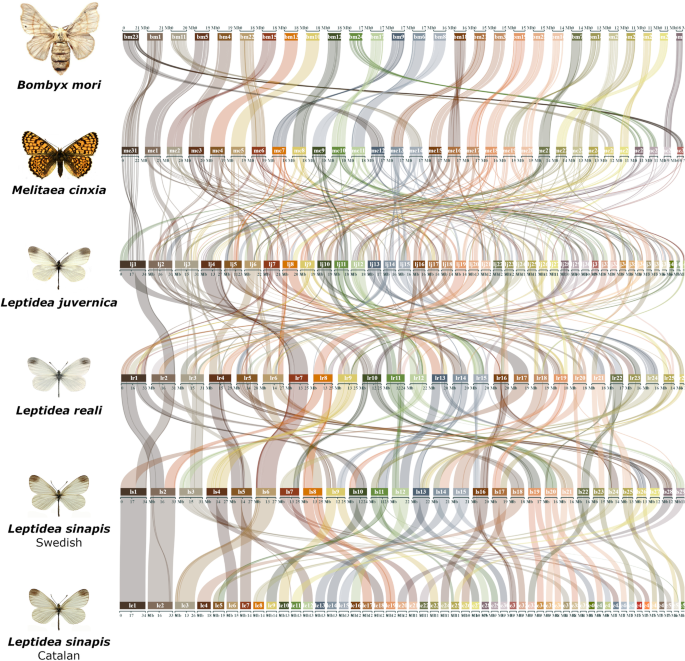The image is an infographic with a white background that features six types of moths on the left, depicted with their Latin names: Bombyx mori, Melitea synxia, Leptidia juvernica, Leptidia reali, and Leptidia synapis (listed twice, once labeled as Swedish and once as Catalan). Each moth illustration is detailed and accurately colored. Adjacent to the moths, on the right-hand side, a vibrant and intricate swirl of rainbow-colored ribbons interconnects various points, paired with numerous small, multicolored rectangles that contribute to a visually striking, almost artistic representation. However, the text within these rectangles is too small to read, making it difficult to discern the specific information being conveyed.